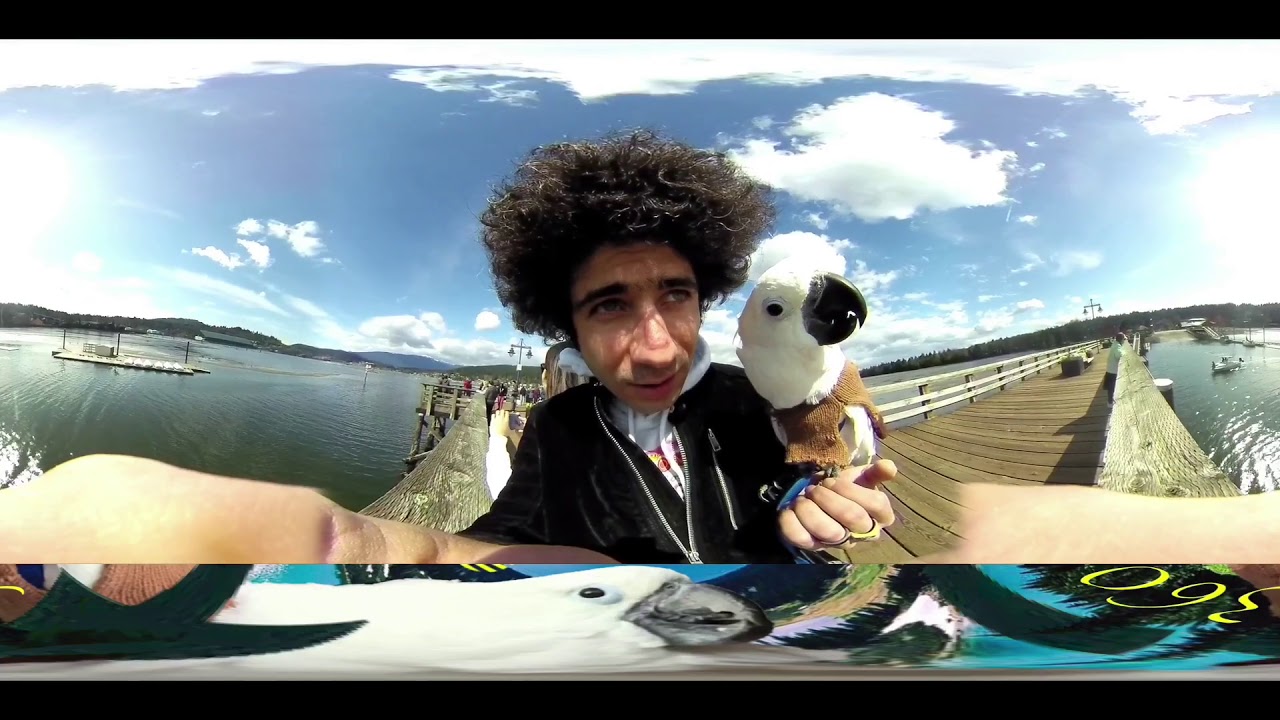The photograph depicts a middle-aged Caucasian man, likely in his 40s, taking a wide-angle selfie. He has a mop of dark curly hair, almost resembling an Afro, dark eyebrows, and is clean-shaven. He is wearing a black jacket with white trim over a white shirt. The man is holding a white stuffed eagle with a black beak in his left hand, bent at the elbow and extended towards the camera. His right hand, partially visible, is holding the camera to capture the shot.

The setting is an outdoor, seaside area with the man standing on a wooden dock that extends backward behind his right shoulder. The scene includes a calm waterway with possibly a marina to his left, featuring several small boats and a flat barge or watercraft in the distance. A rolling hill landmass serves as a picturesque backdrop along with a bright blue sky filled with puffy white cumulus clouds. The sunny day highlights the serene environment and the man's prominent features exaggerated by the close proximity to the camera, including his large nose and deep-set eyes. This color photograph captures a beautifully detailed panoramic view of the scenic waterway and the man's enthusiastic selfie moment.